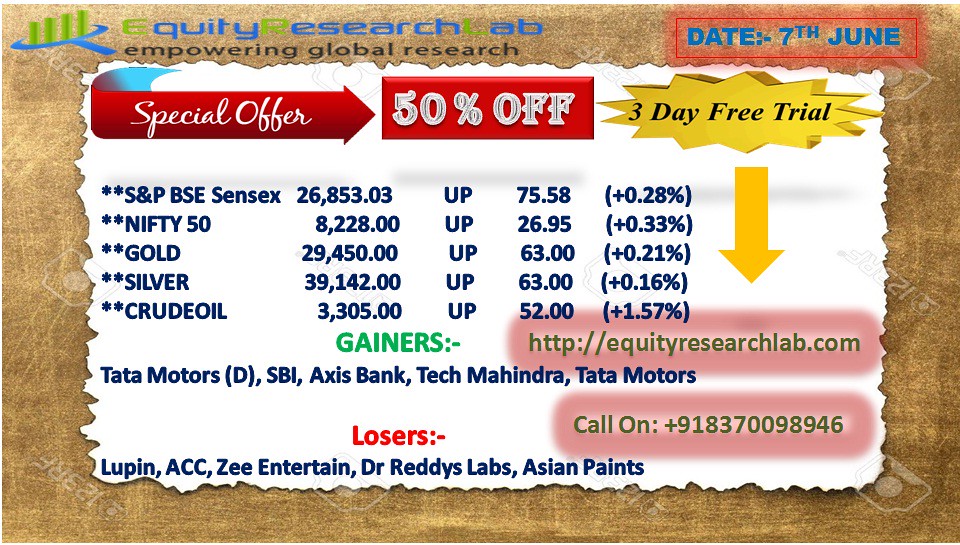This digital advertisement showcases an equity research lab's financial program against a textured, wooden brown background with a white central section bordered by a serrated brown edge, resembling torn paper. At the top of the image, the text "Equity Research Lab: Empowering Global Research" is prominently featured along with the date, 7th June, in the top-right corner. Centrally positioned on the white background, the advertisement highlights a special offer of 50% off a three-day trial, emphasized with red boxes and a yellow star. Financial information is displayed prominently, showcasing an S&P BSE Sensex value of 26,853.03, an increase of 75.58 points (+0.28%). Below this, detailed gainers and losers are listed in green and red respectively, along with other stock and financial data. Contact information including a website and phone number is provided, making it clear that this is a promotional effort by the equity research lab targeting potential investors with a special limited-time offer.